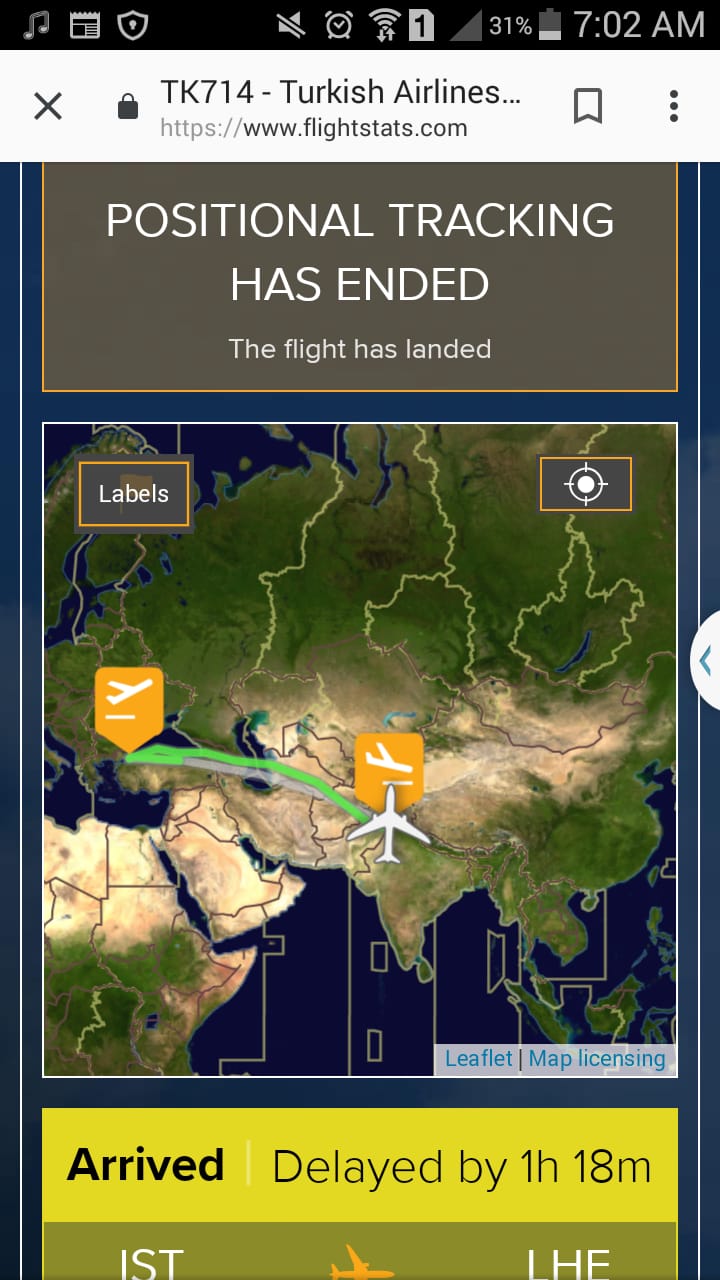The screenshot captures a phone displaying detailed information about a Turkish Airlines flight, TK-714. The phone, at 31% battery and showing the time as 7:02 a.m., has a screen shaped long and narrow. At the top, "Positional tracking has ended" indicates that the flight has landed. Below that notification, a detailed map, colored in green, blue, and beige, depicts the flight's route, showing a white airplane icon mid-route over the region north of India. The map includes a green line marking the flight path. In a yellow bar, it is noted that the flight has "arrived" and was "delayed by 1 hour 18 minutes." The displayed information also mentions that the flight initially took off from a location presumably in Asia, Europe, or Turkey.